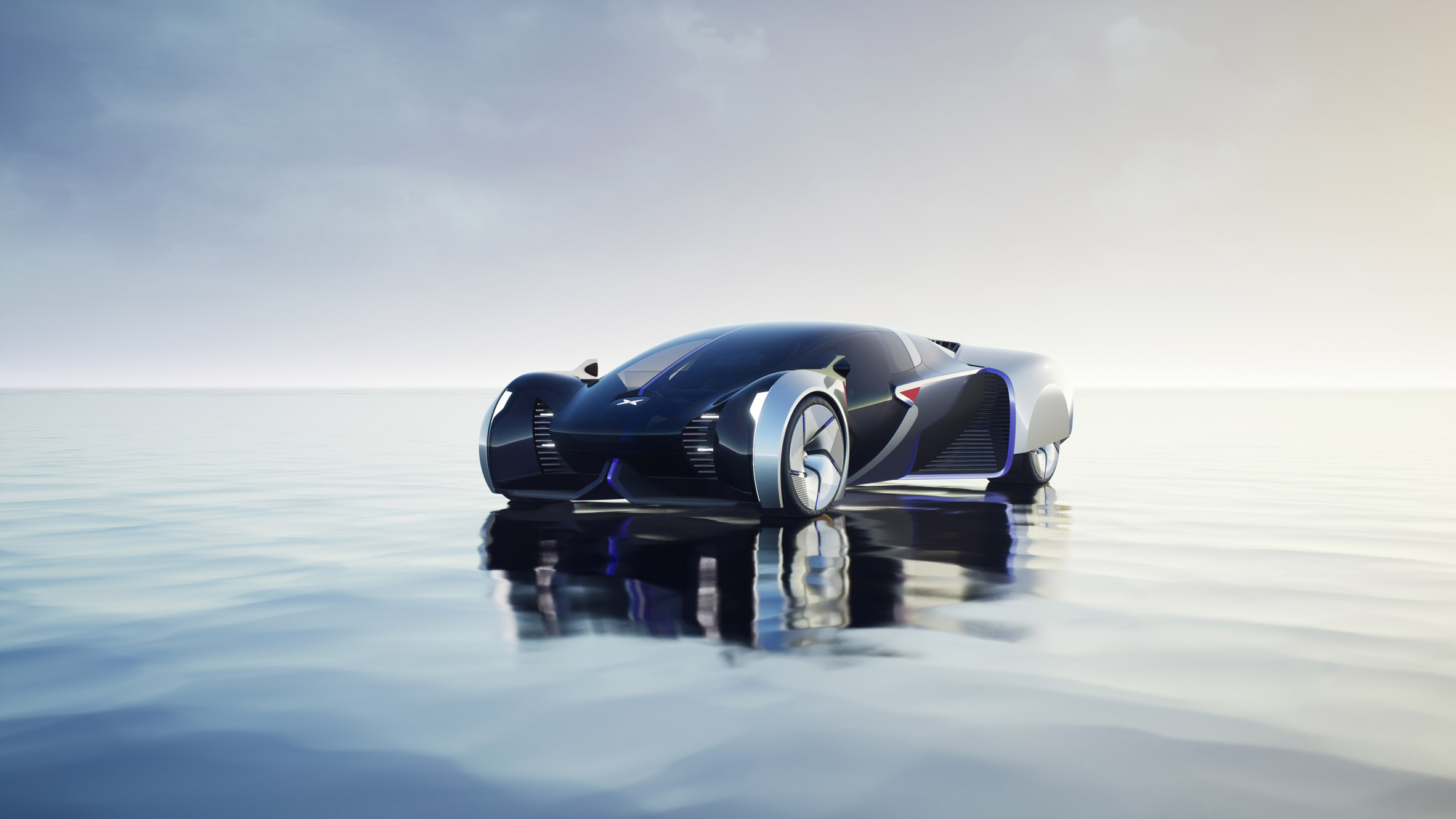The image showcases a horizontally aligned, rectangular picture of a highly innovative and futuristic sports car. The car, sitting atop a gently rippled watery surface that has a bluish-gray hue, is oriented with its front end angled towards the lower left and its back end towards the upper right. The sky above features a blend of blue and white feathery clouds, with a brownish-white tinge on the right side.

This striking vehicle is characterized by its sleek and extremely low profile, with the shell nearly touching the ground. The front end is black and steep, with the hood and front seat nearly at the same height. The rear of the car is primarily gray with a silver finish and features large silver rims. The sides and front of the car sport a purple hue, and the roof is entirely made of glass that likely lifts up for entry. The side mirrors are mounted on the fenders that arch over the tires, designed for aerodynamic efficiency. The rear tires are partially covered by fans extending from the sides, contributing to the car's futuristic, wide stance with large air ducts on the sides indicating a powerful engine. The reflective surface beneath the car, resembling icy ripples, adds to the ethereal and advanced aesthetic of this remarkable vehicle.